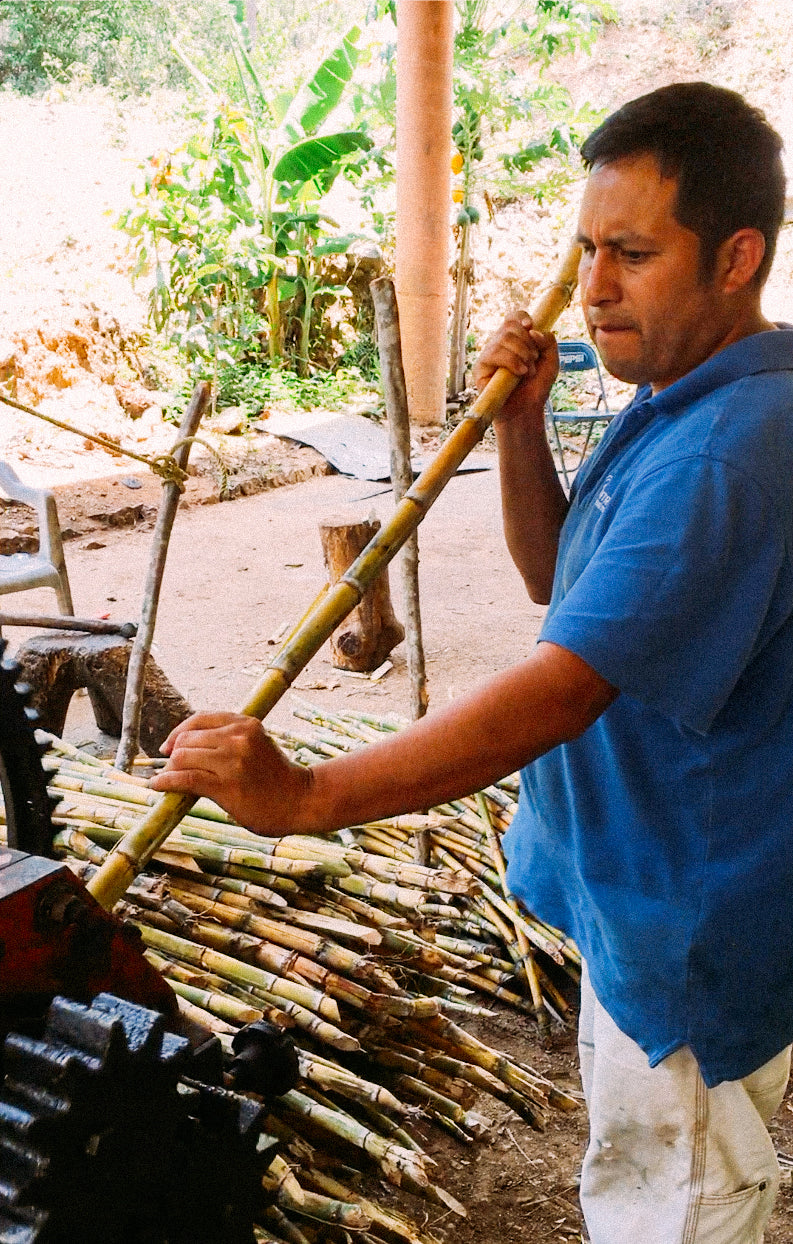In this vertically aligned rectangular photo, a man with short brown or black hair and sideburns is deeply focused on his work, holding a bamboo stick in his hands. He is wearing a blue polo shirt and dirty, beige-colored or white pants, and exhibits a concentrated expression with a slight frown on his face. The man, viewed from his left side, is inserting the bamboo stick into a machine that appears to be for processing or chopping the bamboo, possibly to extract juice. The machine, partially visible at the bottom left of the image, features large black gears and a crank attached to its side.

Beneath and around the man, there is a considerable stack of bamboo sticks, suggesting a significant amount of work or production. The setting of the image is outdoors during the day, featuring a wooden column that supports a probable covered area. In the background, lush green vegetation including bushes, trees, and possibly banana plants indicate a tropical environment. A blue folding chair with some white writing, slightly blurred due to distance, sits to the right of the column. The scene captures the industrious activity in a verdant, tropical locale.